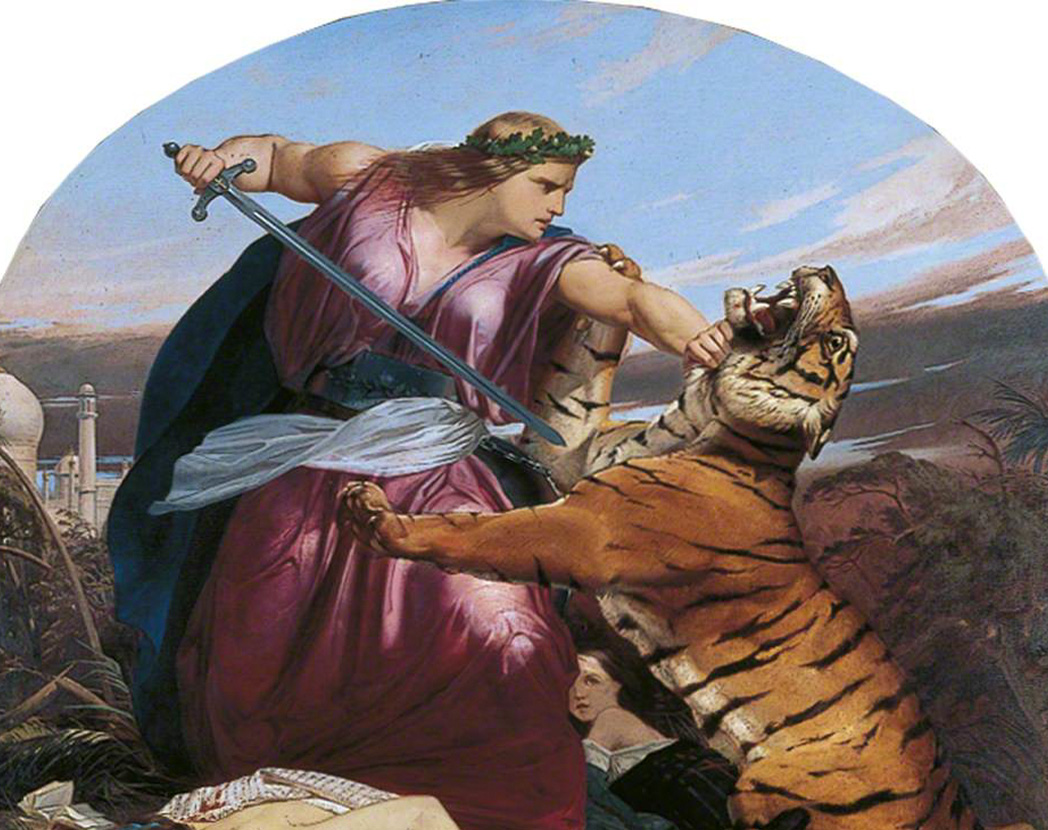This detailed painting features a muscular, warrior-like woman engaged in a fierce battle with a tiger. The woman, facing to the right, boasts a green leaf crown adorning her long blonde hair, emphasizing an ancient or mythological setting. She is clad in a flowing purple dress with a white sash and a dark blue cape billowing behind her, adding to her majestic appearance. Her right hand wields a sword pointed threateningly at the tiger, while her left hand grips the beast's neck with formidable strength.

The tiger, with its orange fur and black stripes, has its mouth open and paws raised—its right paw with outstretched claws resting on the woman's right arm, and its left paw angled outward. Beneath the tiger, a small child with a partially torn white shirt and dark hair is visible, seemingly depicting a scene of protection.

In the background, a cityscape with rounded roofs and towers is faintly visible beneath a blue sky dotted with clouds, adding a sense of depth and place to the piece. The style of the painting suggests an old-fashioned, hand-painted artwork reminiscent of European masterpieces displayed in renowned museums like the Louvre. This fantastical and realistic depiction emphasizes the dramatic and heroic nature of the confrontation.